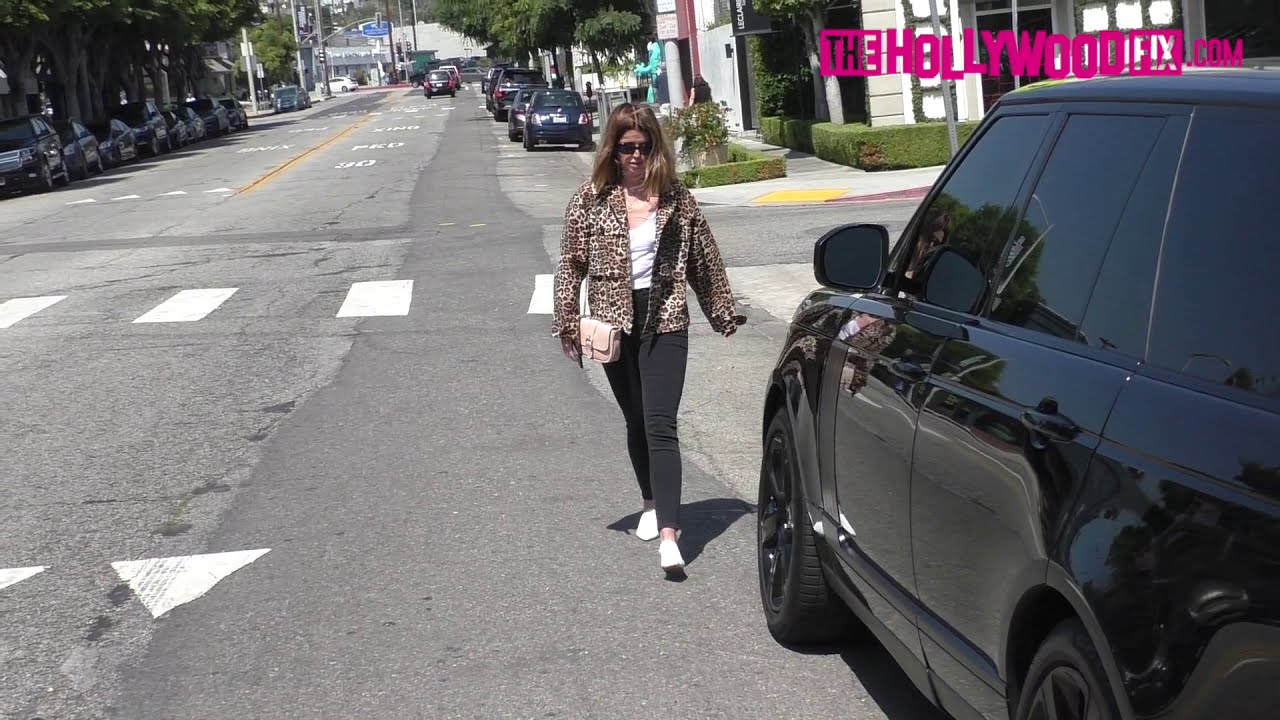In this sunny, paparazzi-style photograph captured on a wide, city street, a woman wearing a leopard print, long-sleeve jacket that ends at her waist stands prominently in the right-hand side of the image. She accessorizes with black pants, white shoes, black sunglasses, and a white purse slung over her shoulder, resting at hip level. Her brownish hair cascades to her shoulders. Adjacent to her, a large black SUV with tinted windows is parked along the side of the road, over which a pink watermark reading "thehollywoodfix.com" is stamped in the upper right-hand corner. 

The street itself features a yellow line down the middle, with a crosswalk visible underfoot. Both sides of the street are lined with trees, parked cars, and various buildings, including a white structure visible in the background. The scene suggests an upscale neighborhood, potentially in Los Angeles or Hollywood, marked by the presence of street signs and the vibrant colors of the surroundings: black, brown, white, green, pink, blue, yellow, and gray. The woman is captured mid-step, seemingly heading towards the black SUV, with a backdrop of urban elements that include more parked cars and a variety of buildings stretching down the left and right sides of the street.